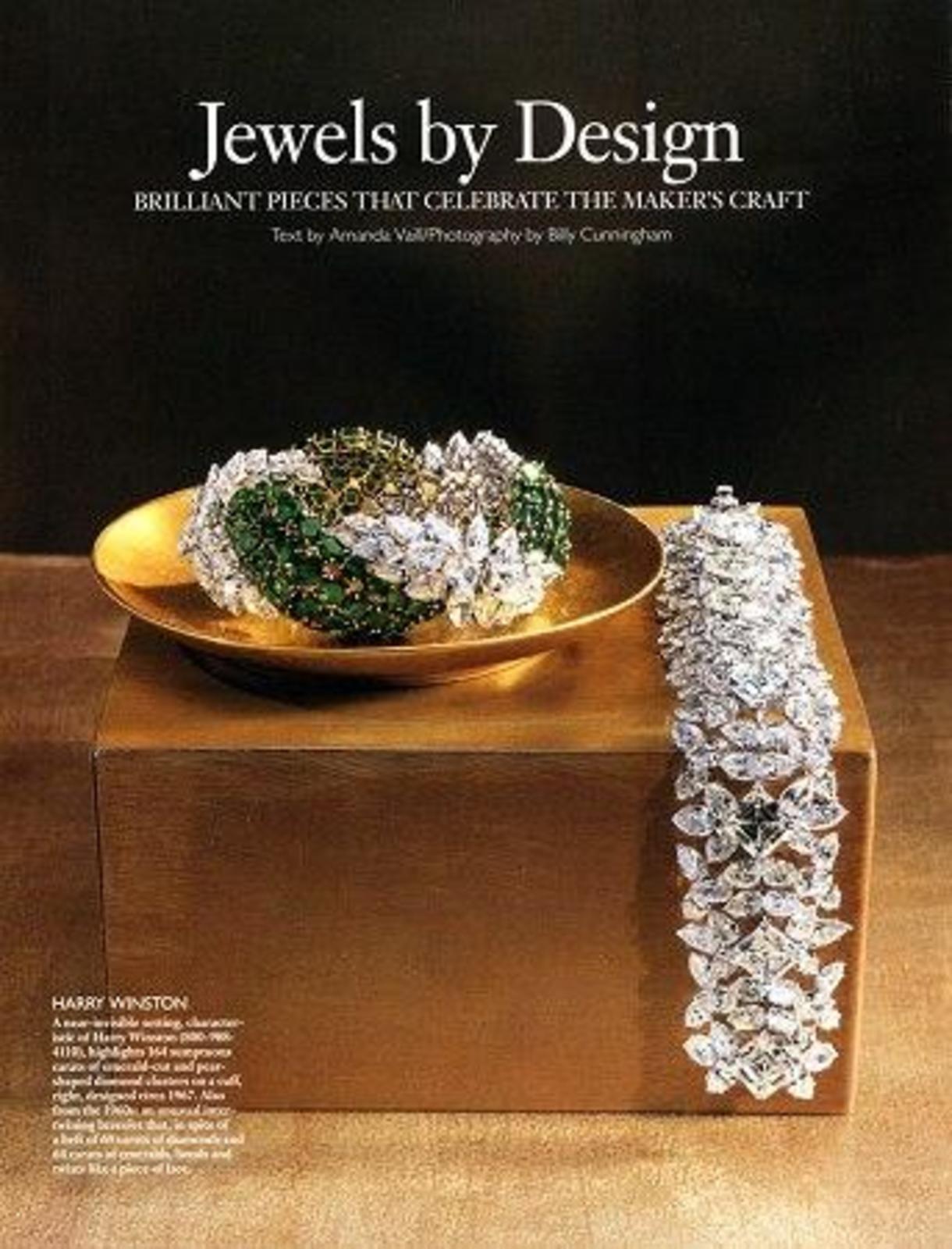The advertisement features a meticulously crafted presentation of luxurious jewelry set against a stark black background. At the top, in elegant white lettering, it reads, "Jewels by Design: Brilliant pieces that celebrate the maker's craft." A gold square ottoman or display block sits prominently in the center, draped with an exquisite array of petal-shaped jewels, possibly from an opened clasped bracelet, cascading over the top and down the side. Positioned centrally on the block, a shallow gold dish holds a stunning, ornate cuff bracelet encrusted with green jewels and diamond-like stones encircling its entirety. To the right, another diamond bracelet, designed in floral motifs, is elegantly laid out on the gold block. The bottom left corner of the image bears the name "Harry Winston," followed by additional promotional text. The photograph credits text to Amanda and photography to Billy Cunningham, enhancing the ad's polished and sophisticated presentation.